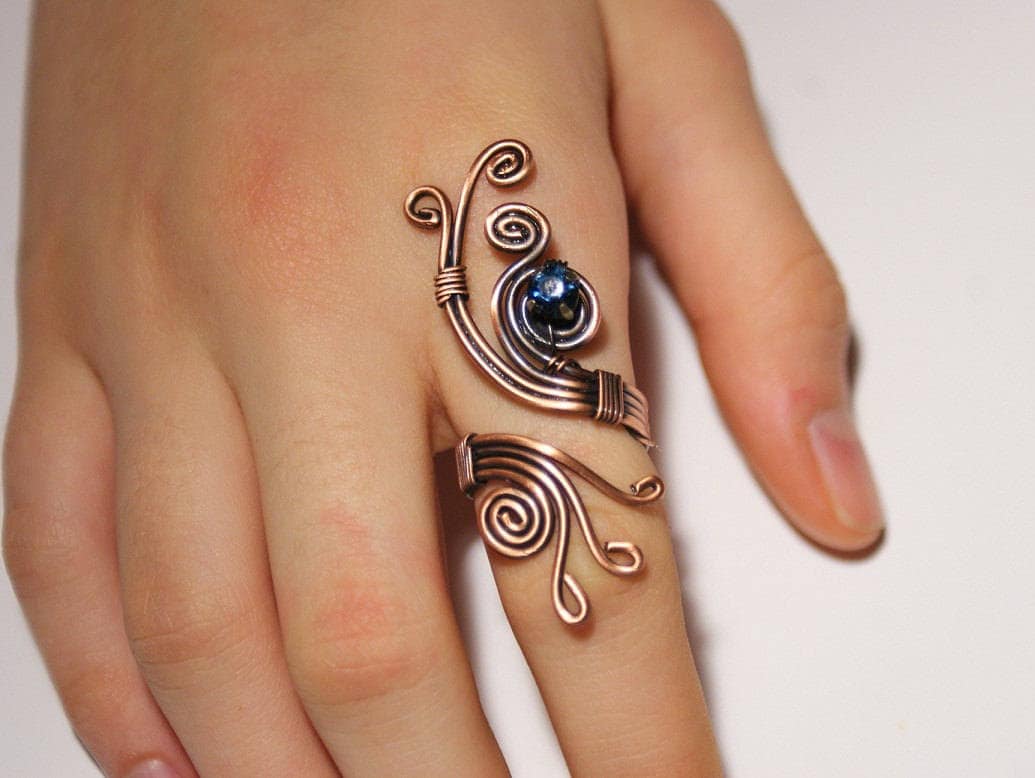The image features a close-up shot of a young woman's hand, resting palm down on a white tabletop. Her light-colored thumb is positioned towards the upper right, while her pinky extends towards the bottom left. On her index finger, she wears an ornate and elegant ring crafted from twisted copper wires. These wires are intricately shaped, forming spirals and small tight circles that reflect light beautifully, appearing very clean and polished. At the center of the ring's design sits a dark blue gemstone, likely a sapphire, which is tightly entwined in the copper wire. The ring is an elaborate piece with the copper wires fanning out towards the ends, creating a swirly pattern that adds to its decorative and sophisticated allure.